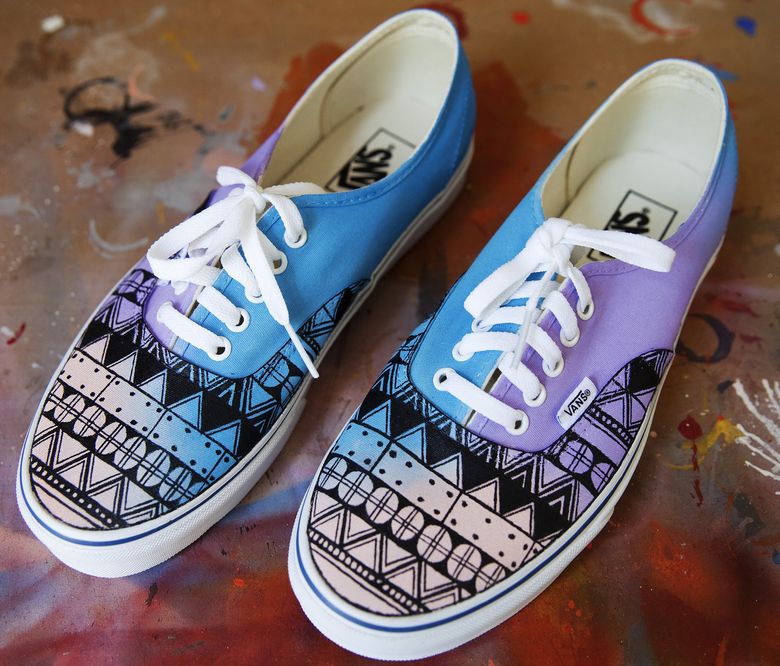This image features a pair of low-cut Vans slip-on sneakers adorned with a vibrant, repeating pattern of plaid circles, triangles, rectangles, and other geometric symbols in black and white. One shoe is predominantly purple on one side and blue on the other, while the opposite shoe has the reverse color scheme. Both shoes have white laces and white soles bordered by blue. The interior displays the Vans logo. The shoes rest on a highly painted surface featuring a collage of red, blue, white, and orange spray paint splotches, adding a dynamic background to the pristine, never-worn sneakers.